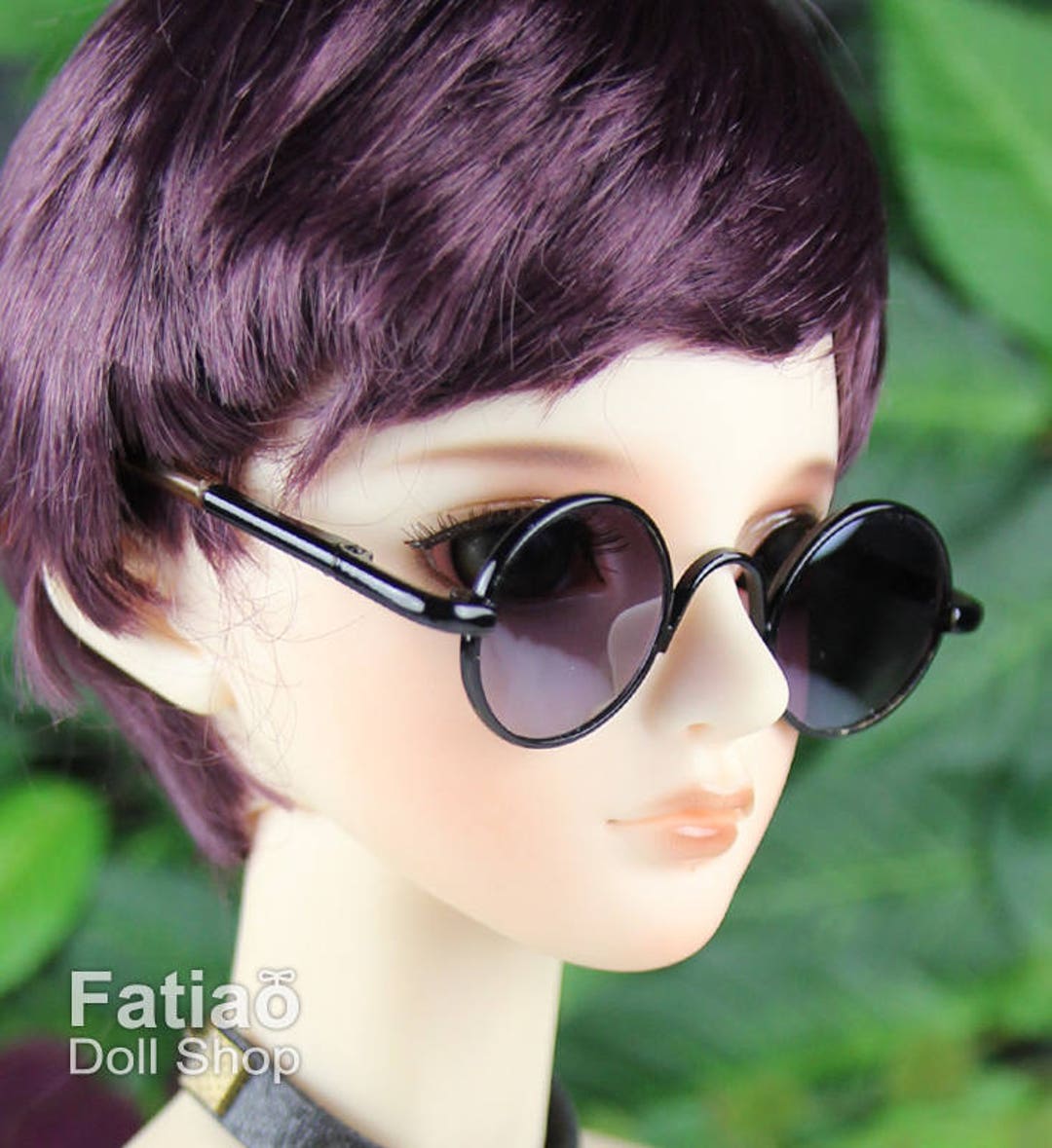This photo depicts a cartoonish doll or mannequin, likely used for advertisement, with an intricate appearance and a backdrop of slightly blurred green foliage. The doll has striking, dark purple hair with a slight gradient hinting at black, beautifully highlighted by the lighting. Its hair falls just past the ears and down to the neck. The doll's face features prominent details: long eyelashes, thick irises, and a subtle application of mascara, along with red blush on the cheeks and pinkish-red lips shaped into a slight smirk. The doll is accessorized with round, black-rimmed sunglasses that have dark purple lenses mirroring the color of its hair. Additionally, the doll wears a stylish necklace with a symbolic design. In the bottom left corner of the image, white text reads "F-A-T-I-A-O" followed by "Doll Shop," indicating it may be tied to an advertisement for the Fashio Doll Shop.